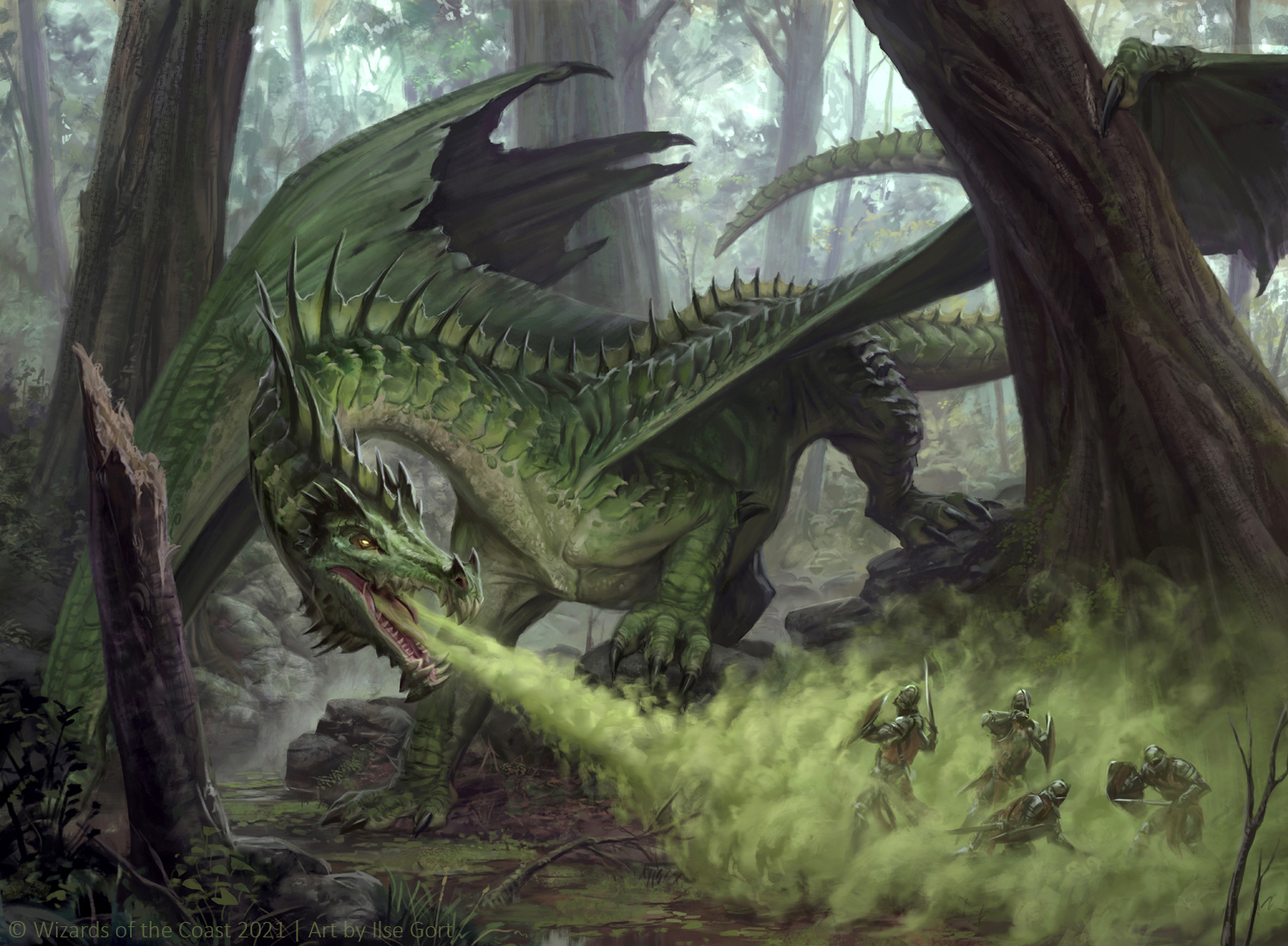The image is a highly detailed, computer-generated scene resembling a moment from an intense fantasy video game or science fiction movie. It depicts a large, green dragon with a spine lined with sharp spikes and long, curving wings. The dragon stands in the middle of a dense forest, surrounded by twisty and turny tree trunks that reach upwards with vibrant green leaves, partially obscuring a cloudy, gray sky. With gold eyes gleaming, the dragon has its head turned back towards the lower right corner of the image, exhaling a massive cloud of greenish-gray smoke or gas.  

On the receiving end of this fierce attack are four warriors, each equipped with shields raised in a desperate bid for protection. They are clustered together, with one visibly turning around, striving to fend off the dragon's powerful breath. The scene emphasizes the overwhelming power and imposing presence of the dragon compared to the outmatched warriors. The illustration features a palette of light and dark greens, browns, off-whites, blacks, and tans, emphasizing the natural, yet otherworldly atmosphere of the forest setting.